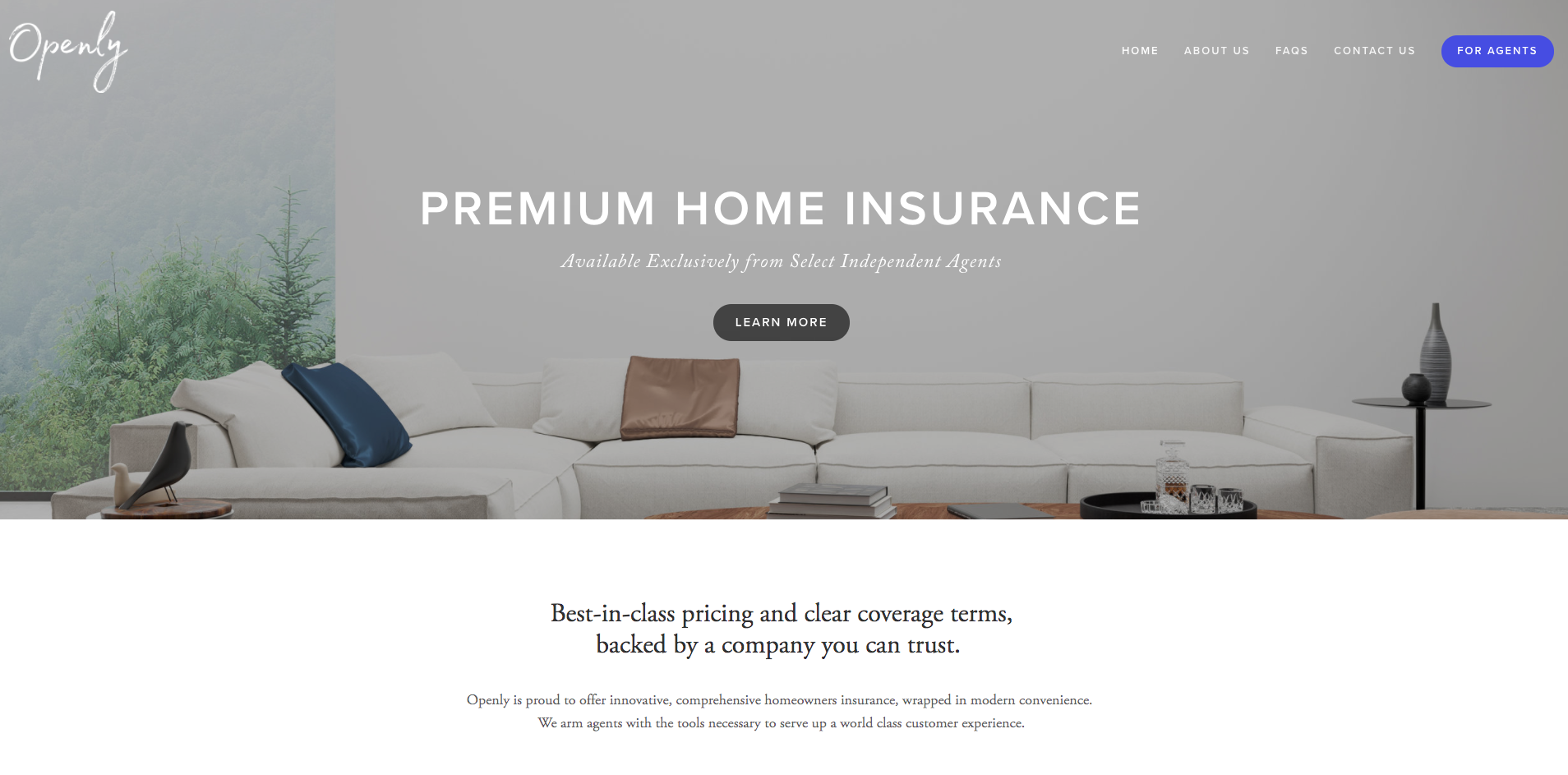This appears to be a promotional email or a website mock-up, primarily featuring a white background. The top half of the image is dominated by a horizontal banner showcasing a stylish living room. The room highlights a spacious L-shaped couch adorned with a variety of pillows, including one in a gold shade and another in navy blue. A painting portraying trees and a dimly visible mountain adds an artistic touch to the background. 

In the living room, there are small circular tables decorated with bottles, vases, random ornaments, and stacks of books, adding to the cozy atmosphere. Overlaying the banner image is the text "Premium Home Insurance" in bold white letters. Directly below, a dark gray "Learn More" button features white text, inviting further exploration.

In the upper left corner of the banner, the word "Openly" appears in cursive, acting as a logo. To its right, the navigation bar in white text includes "Home," "About Us," "FAQs," "Contact Us," and a blue button labeled "For Agents."

Below the banner, the white background continues with black serifed text that reads, "Best-in-class pricing and clear coverage terms, backed by a company you can trust." Following these details, there are additional sentences in low-resolution text that are difficult to decipher.